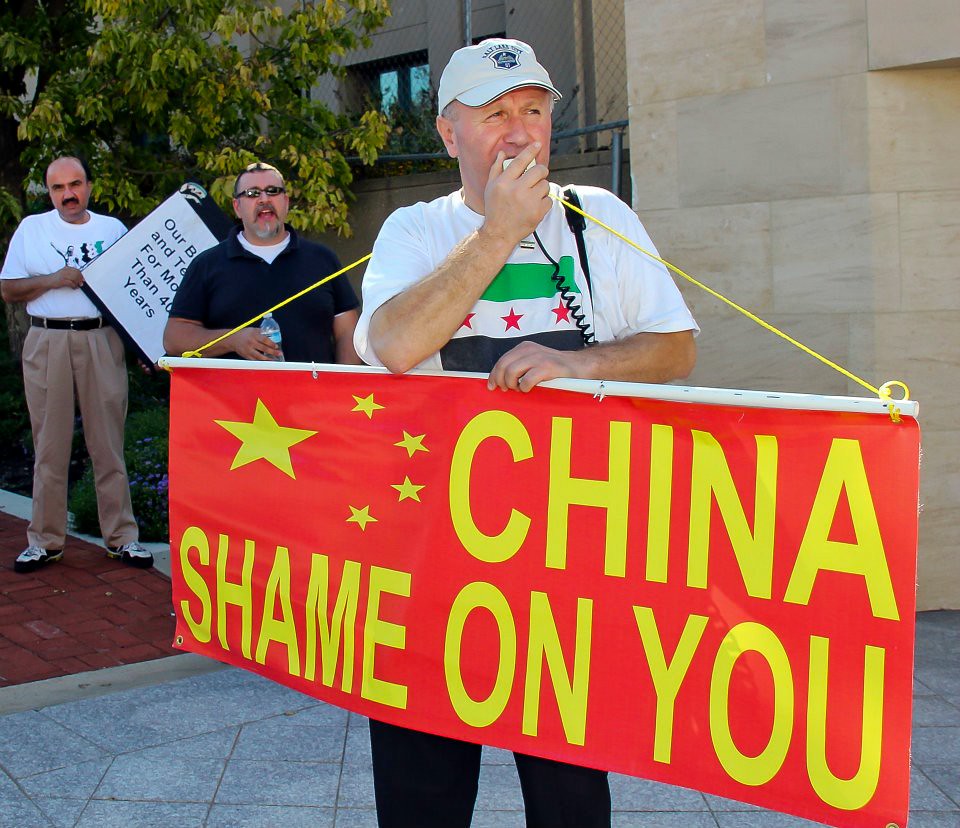This image features an outdoor protest scene in front of a building with tan tile siding. At the forefront stands an older man wearing a white baseball cap and a white t-shirt with a flag emblem, speaking into a microphone. He's holding a large red banner with bold yellow letters that read, "China, shame on you." The pavement below him includes both red and gray bricks. Behind him, two other men are present. The man directly behind him wears sunglasses, a black short-sleeve t-shirt, and holds a water bottle. The third man, positioned farther back, is dressed in a white t-shirt and khaki pants, holding a partially obscured sign that reads something along the lines of "our [blank] for more than 40 years." A small tree with visible leaves and a brick-paved area complete the background.